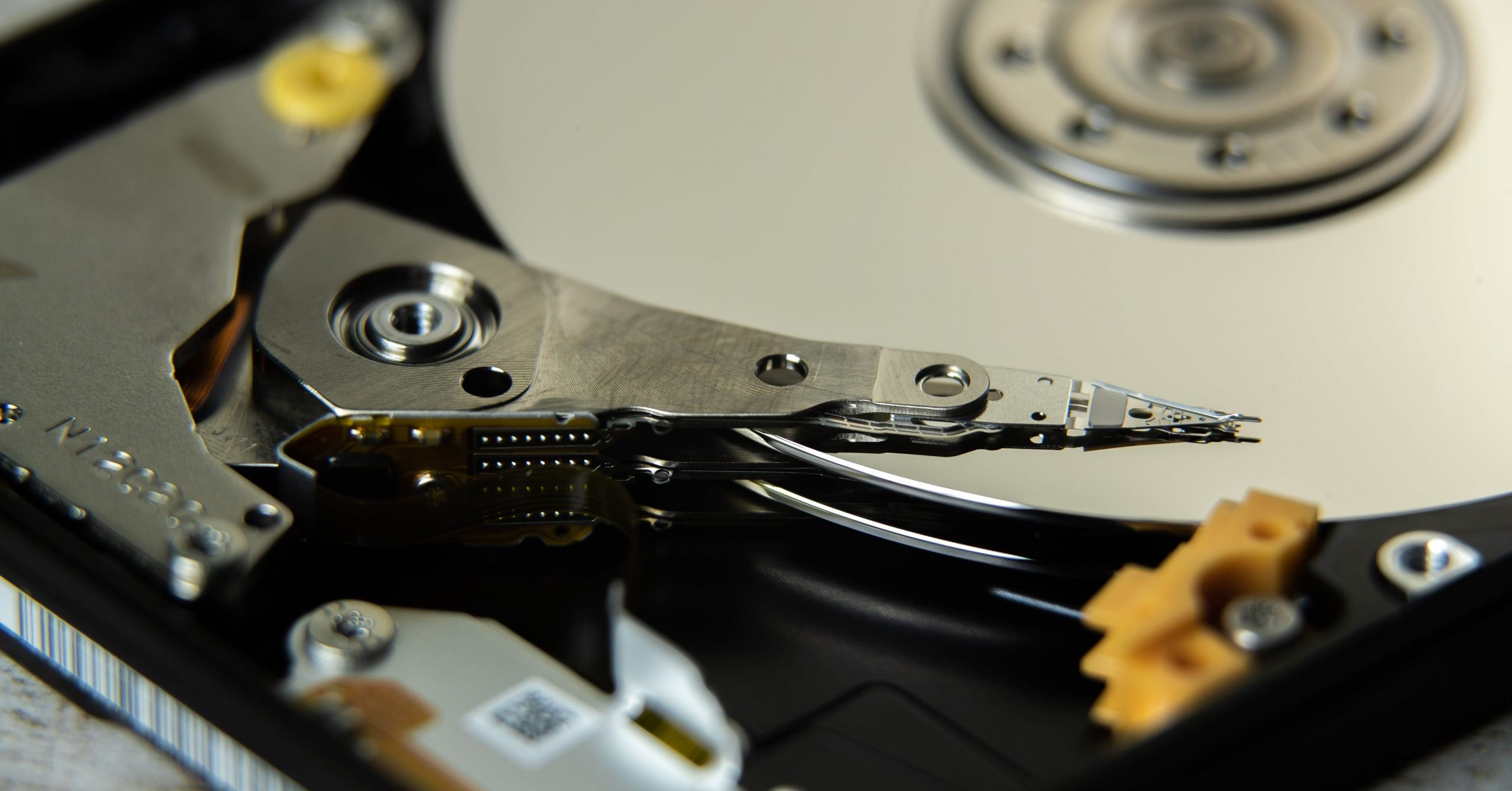This detailed close-up image showcases the intricate interior of a hard drive. Dominating the right side of the image is a large silver magnetic disk, featuring a smaller, elevated circular structure at its center with multiple connections. To the left of this disk, a precisely-engineered metal arm extends over the magnetic surface. The arm culminates in a sharp, arrowhead-like point and is attached to a steel triangular component inscribed with numbers and letters, likely "N120" or "21," near a distinctive screw. Adjacent to this, a brown metal piece with rows of stainless steel dots and two prongs is also secured with a special screw. The housing of the hard drive is built from shiny black plastic, with contrasting yellow plastic tabs situated near silver screws providing additional connection points. The left edge of the mechanism features a white strip with a barcode, completing the complex assembly depicted in this micro-view.